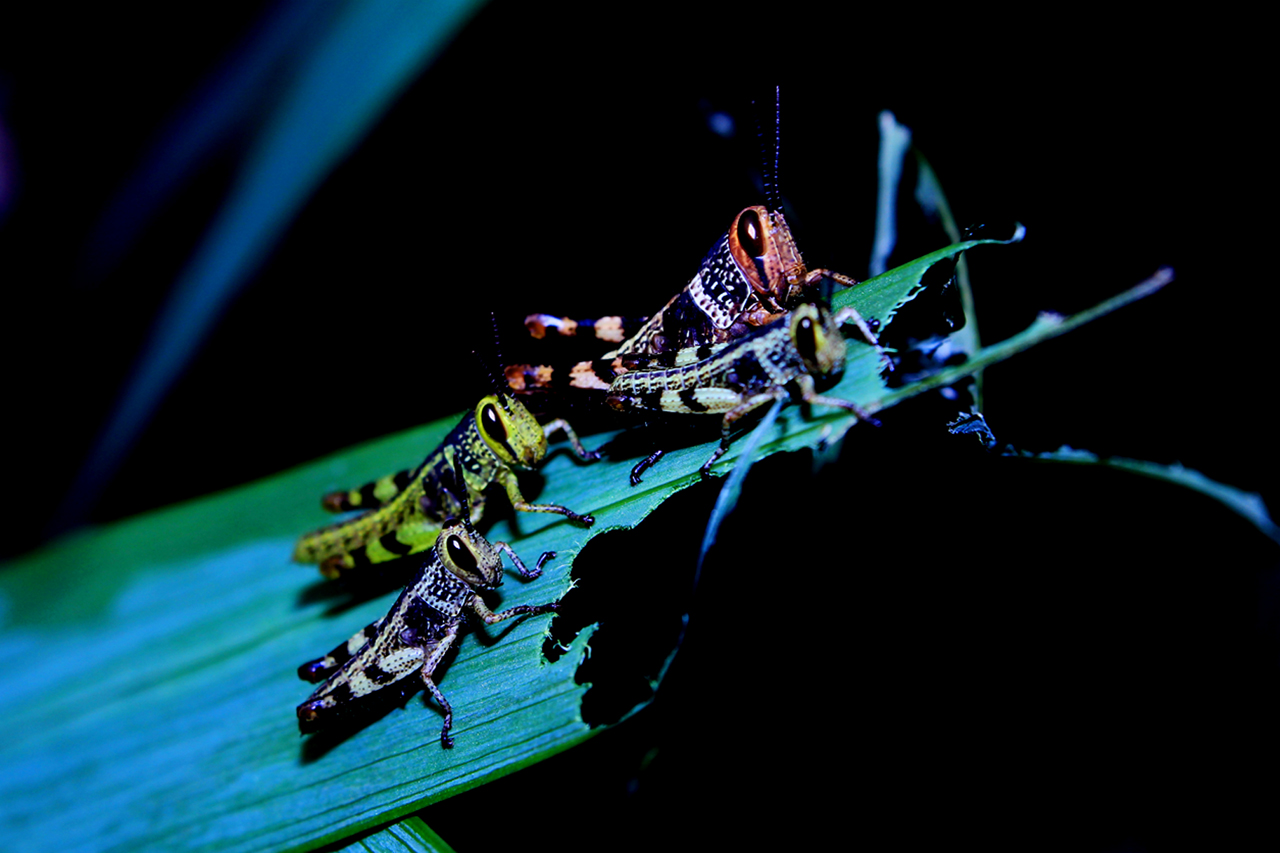This photograph captures a fascinating close-up of four distinctively colored grasshoppers perched on a long, wide green leaf against a dark, night-time background. Each grasshopper's unique appearance and vibrant hues are strikingly highlighted by subtle moonlight, revealing a palette of bright colors—one is predominantly orange, another is yellow, a third is green, and the fourth has a dark, almost black body with a few white spots and a green-tinted head. All of them feature black markings that contrast sharply with their vivid exoskeletons. The leaf they are sitting on is visibly being consumed, with clear and detailed bite marks and circular indentations showing their feeding activity. The largest grasshopper displays an orange and brown coloring, while the medium-sized ones exhibit more green tints. This nocturnal setting enhances the intrigue of the scene, emphasizing the grasshoppers' vibrant colors against the stark blackness of the background.